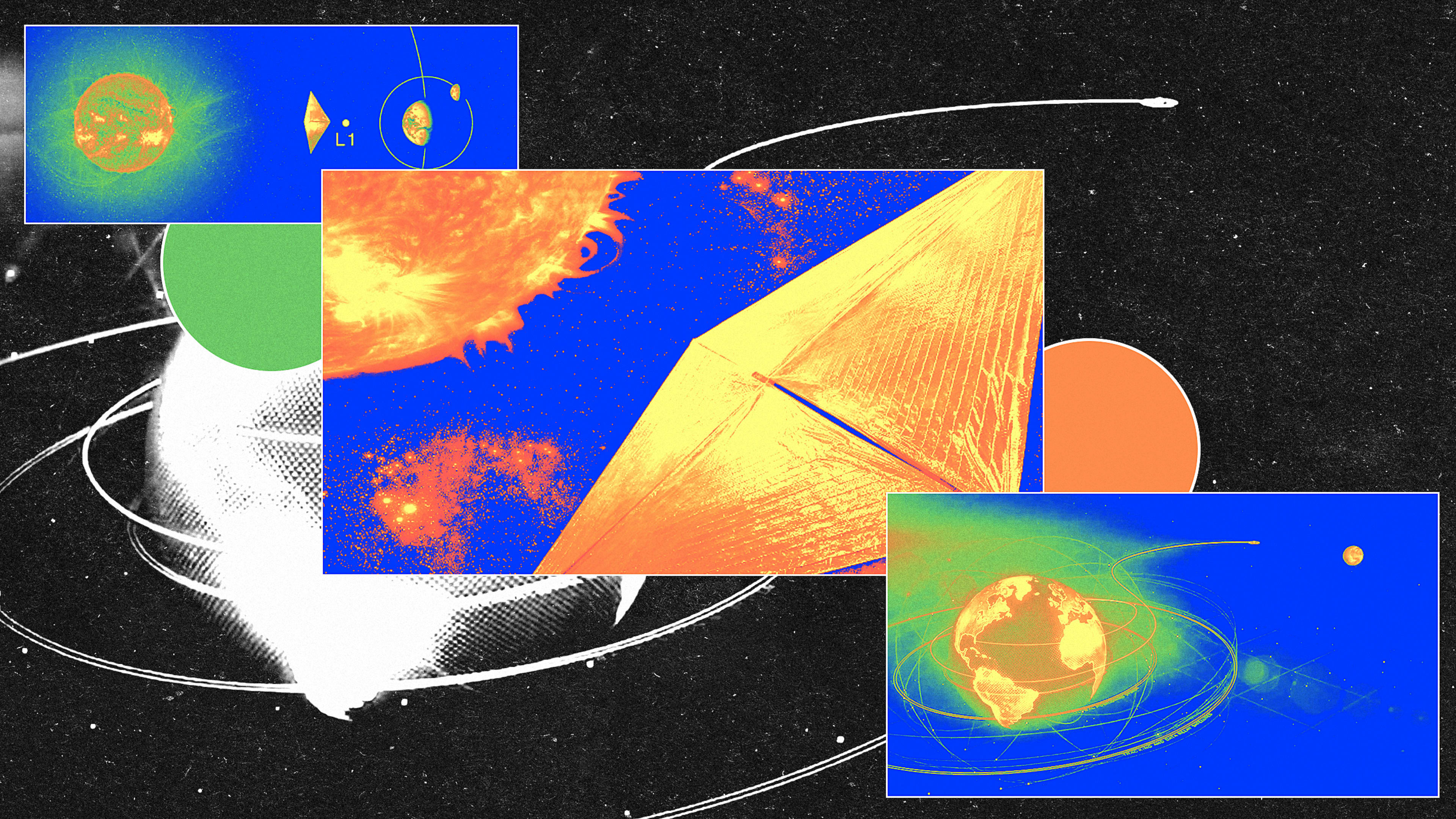This composite image depicts a detailed scene of outer space with a central focus on the sun and Earth, set against a black backdrop scattered with white stars and swirling patterns. There are three smaller rectangular images overlaid onto the background:

1. **Top Left Rectangle**: Features a zoomed-out view with a blue background. An orange Earth with a glowing green mist surrounds it. To the left of Earth is a yellow kite-like shape labeled "L1". Above and to the right of Earth is a partial view of the sun.
   
2. **Center Rectangle**: Positioned slightly above and overlapping the bottom-left corner of the first rectangle, it has a close-up of the sun depicted in orange against a blue backdrop. An orange kite-like shape hovers in the bottom right corner of this rectangle.
   
3. **Bottom Right Rectangle**: Partially obstructing the bottom corner of the central rectangle, this image also showcases the Earth highlighted in orange with a green mist, set against a blue background.

Additionally, peeking out between the overlapping images, we see small circles: an orange circle to the right and a green one to the left, adding depth and complexity to the overall composition. The depiction of kite-like figures could symbolize observational devices used to study these celestial bodies.